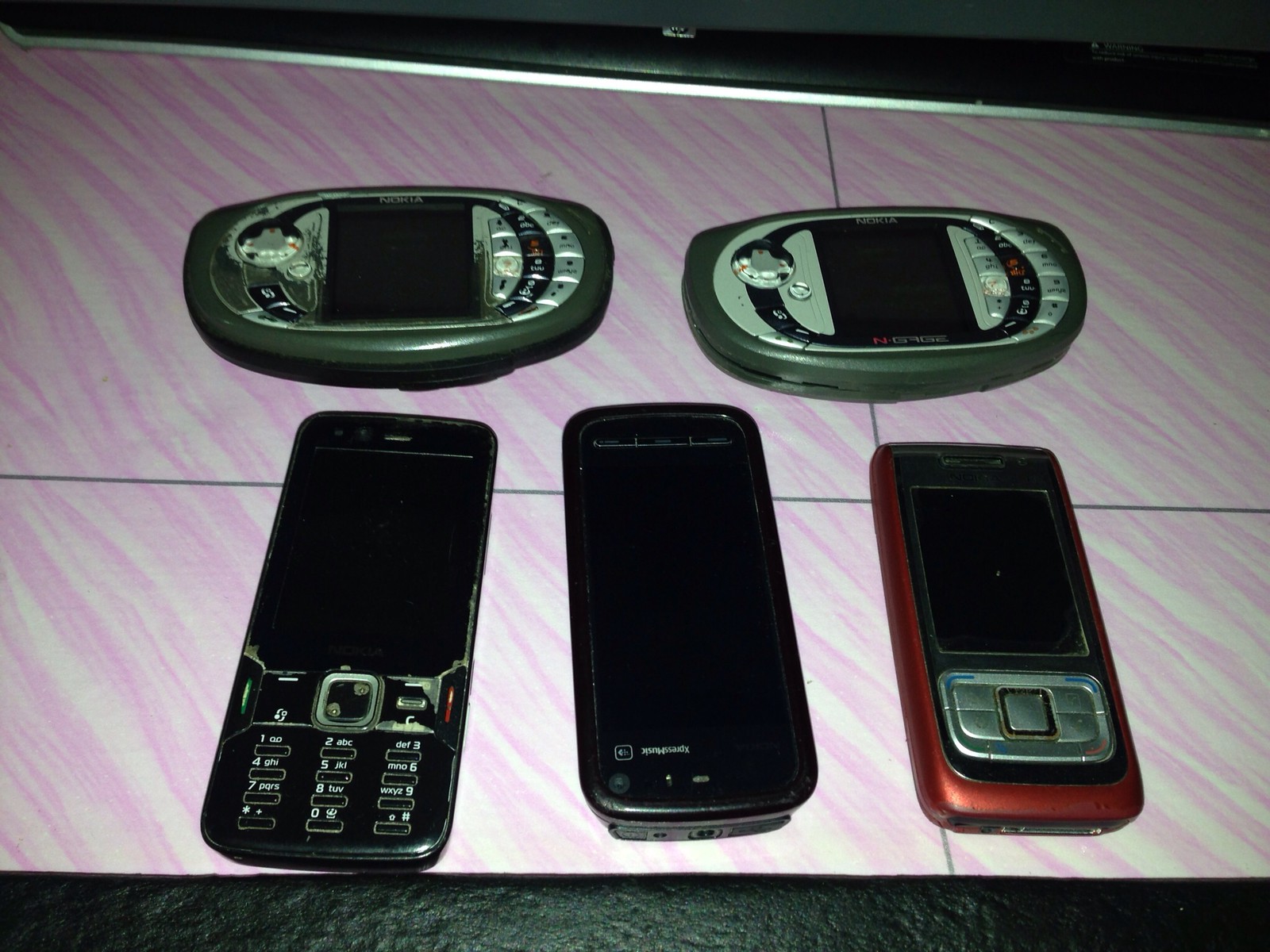This detailed photograph captures a close-up of a multi-colored table or surface with distinct black edges at the top and bottom, and a pink-striped central section. The tabletop features diagonal stripes in various shades of pink, bordered by dark lines. Positioned on this surface are five old-fashioned mobile phones, suggesting the image has historical significance.

At the top, there are two horizontally oriented devices resembling early 2000s Nokia phones, characterized by small, nearly square screens and physical keypads. These may evoke memories of early texting-centric devices akin to BlackBerrys. Below them, three vertically aligned phones, likely from the 2010s, rest side-by-side. The two phones on the left are black, while the one on the right features a distinctive red frame around a black center. 

Detailed observations reveal that one phone has numeric keypad buttons similar to those on a calculator with white text labeling each key, while another features five metal buttons positioned beneath a smaller screen. The devices showcase a range of antiquated designs, encapsulating a nostalgic glimpse into the evolution of mobile technology against a visually striking background.